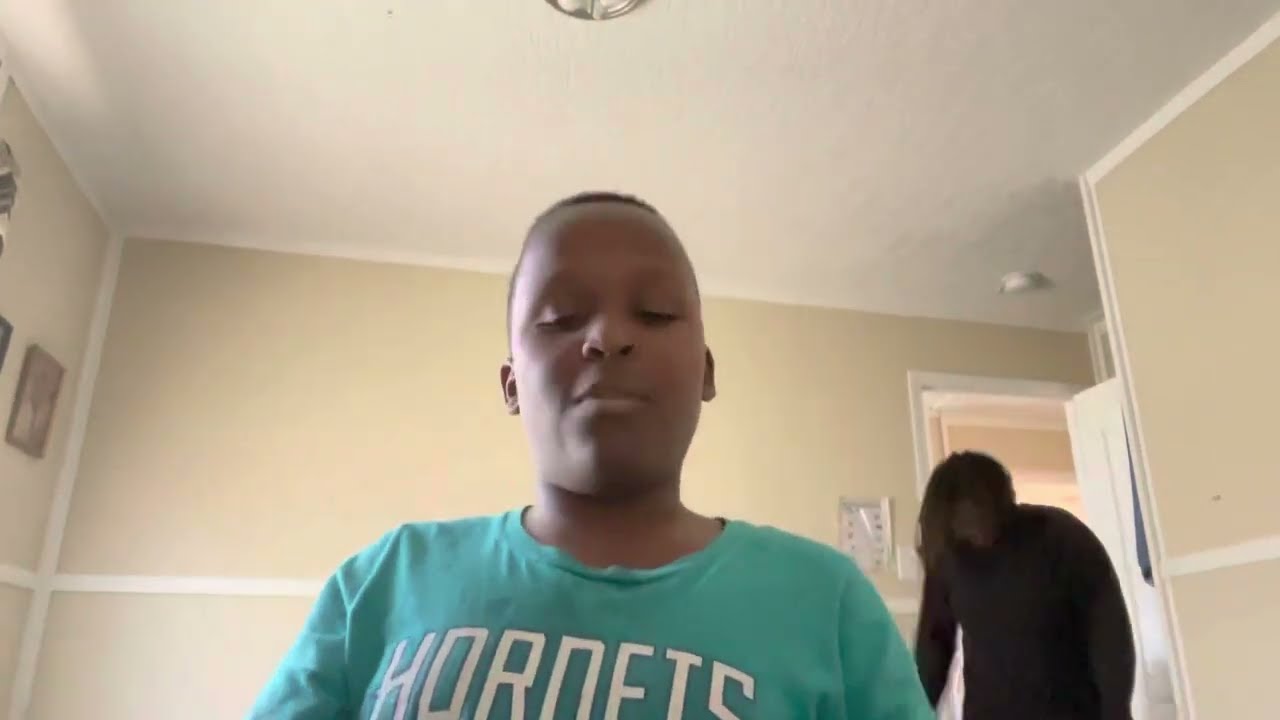This indoor photograph features a young African-American teenager positioned at the center, wearing a blue t-shirt with white text that likely reads "Hornets." The teenager, whose eyes are closed or looking downward, appears motionless, perhaps caught in a moment of reflection or concentration. To the right, partially behind the teenager, is a blurred figure – possibly an older male, dressed in black, with their head also angled downwards. The setting appears to be a room with cream-colored walls and a white ceiling. On the left wall, several paintings or pictures are displayed. Above and behind the blurred figure, an open door and a smoke alarm on the ceiling are visible, adding context to the indoor domestic environment. Light softly illuminates the scene, contributing to a calm, introspective atmosphere.